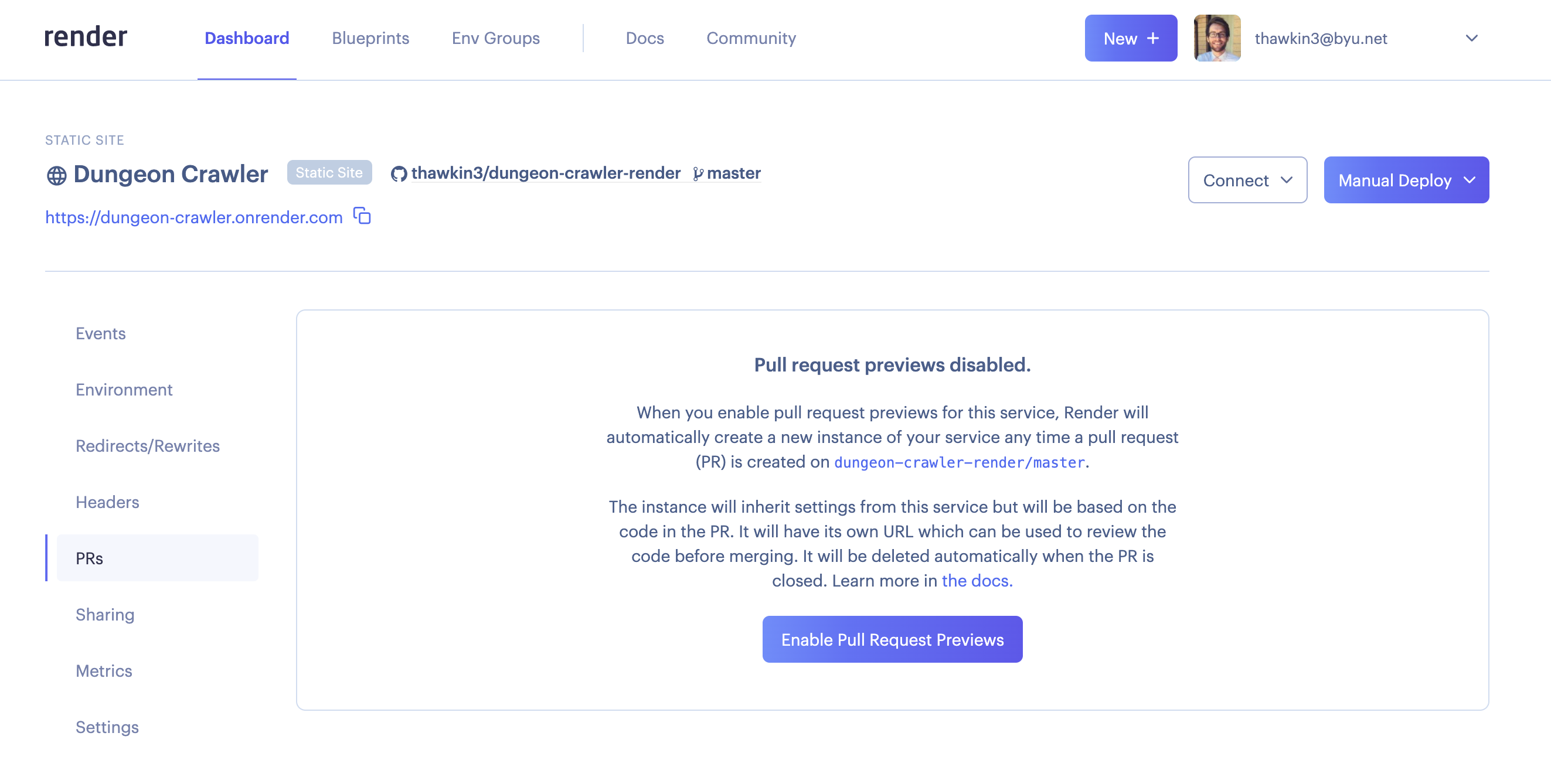The image captures a screenshot of a website interface for a service called Render. In the top-left corner, the word "Render" is prominently displayed in black. Adjacent to it, the section labeled "Dashboard" is highlighted and underlined in blue, indicating the current page. Other menu items listed include "Blueprints," "ENV Groups," "Docs," "Community," and "New," the last of which is housed in a purplish-blue box accompanied by a plus sign.

On the upper right side, a user's profile image is visible. The individual depicted has black hair and appears to be wearing glasses. Their username is also displayed.

Central to the interface is information related to a static site named "Dungeon Crawler," with its URL specified as "DungeonCrawlerOnRender.com" in blue. Below this, a purpley-blue button labeled "Enable Pull Request Previews" stands out.

A box situated in the middle of the page features a message stating "Pull Request Previews Disabled." The text elaborates that enabling Pull Request Previews will prompt Render to automatically create a new instance of the service upon the creation of any Pull Request (PR) on "DungeonCrawlerRender.com." This instance will inherit settings from the original service but will be based on the code in the PR. Each instance will also receive its own unique URL for code review before merging and will be deleted when the PR is closed. Further information can be found by clicking the "Learn more in the docs" link.

On the left side, a vertical menu displays various sections including "Events," "Environment," "Redirects," "Rewrites," "Headers," "PRs" (which is highlighted with a purpley-blue bar), "Sharing," "Metrics," and "Settings." Additionally, the PR section is emphasized by a shaded box.